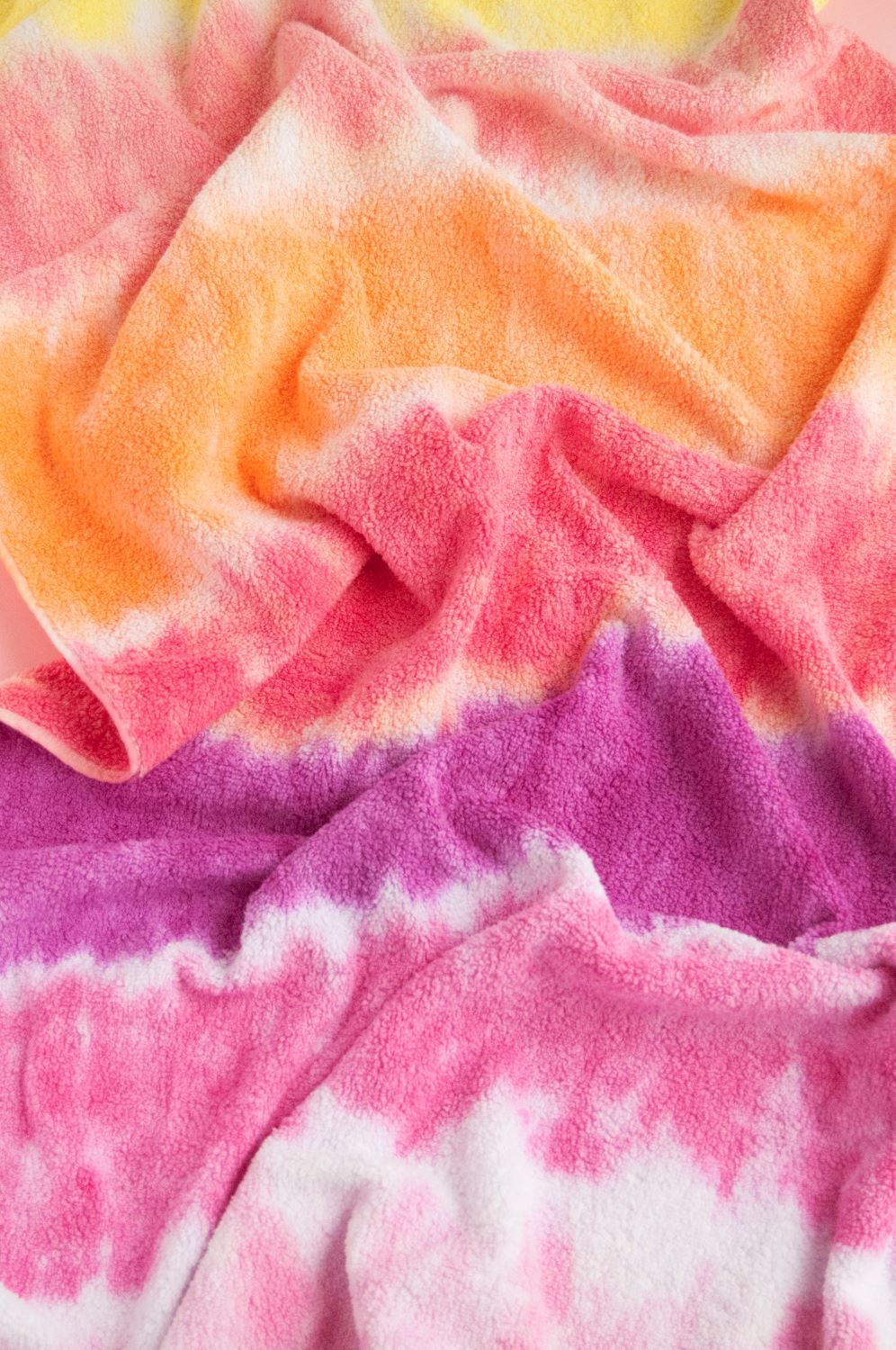The image showcases a vertically-oriented, slightly crumpled tie-dyed towel laid across a surface. The towel's vibrant colors transition in a striped gradient, starting with a pale yellow at the top, followed by sections of salmon pink, fresh orange, darker pink, a pinkish-purple, raspberry pink, and ending in a light bubblegum pink. White fuzzy stripes separate each block of color, typical of a homemade tie-dyed pattern. The towel features numerous folds and creases, giving it a textured appearance, and the creases in the center form a mountain-like shape. A small part of the white table beneath is visible at the middle left of the image. The overall composition is dominated by the towel, with no other elements or text present, capturing the intricate details and shadows of the fabric in a close-up shot.